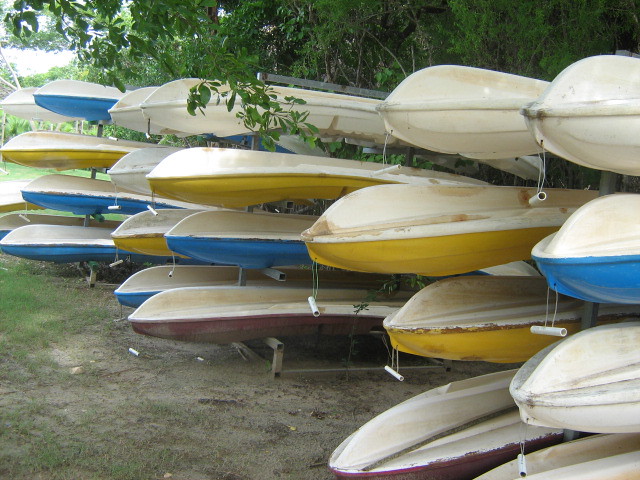The color photograph, taken outdoors in landscape orientation during daylight, captures an organized storage area filled with numerous canoes stacked upside down on gray metal racks. The canoes, vibrant in their colors—bright yellow, magenta purple, aqua blue, white, and some brown—are arranged in rows, typically stacked four high. The racks form distinct metal shelving structures that hold the canoes securely. The bottoms of the canoes face upwards, showing signs of wear and usage, with visible skid marks indicating their frequent handling. 

In the background, large trees with green foliage cascade over the canoe stacks, partially draping down and framing the scene, though the tops of the trees are cropped out of the image. The ground, predominantly light gray and brown earth color, is heavily worn from repeated use, interspersed with a few patches of grass snaking along the left side of the image. The storage area appears well-used and possibly part of a marina, likely serving as a rental facility.